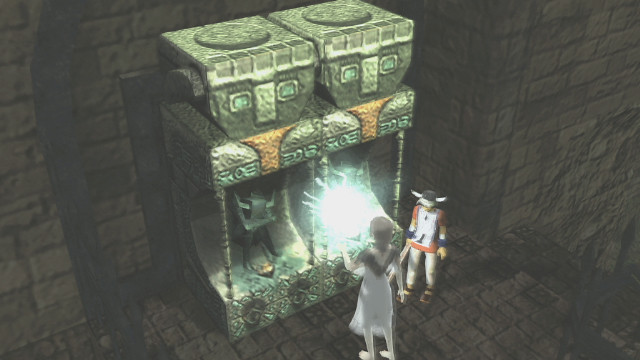This image appears to be a screenshot from an isometric, top-down computer game set in a dark, castle-like environment filled with grey, brown, and dull horizontal bricks. At the center of the scene stand two abstract, cubic rectangular statues side by side, made of darker gray stone with lighter gray tops that feature a round identical area. The statues have neon-colored eyes and a lighter gray area resembling a nose between them. Just below their chins, there’s a funnel-like section with an orange, stony texture.

In front of these statues is a girl with dark hair, barefoot and wearing a white dress. She appears to be holding a blindingly bright, white ball of light in her hands. Next to her stands a younger boy wearing a baseball hat adorned with white horns, a red shirt covered by a white apron-like garment with the number one on it, and light pants. The ambiance suggests a gothic or underground setting, enhancing the eerie, mystical atmosphere of the image.